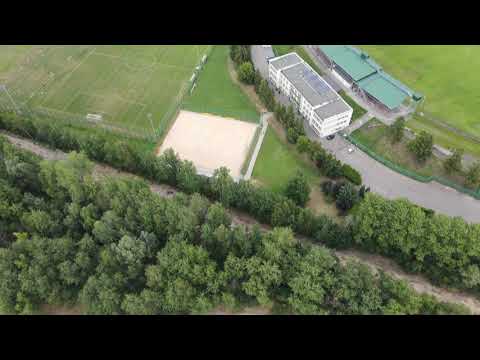This aerial photograph captures a vast sports complex that centers around a large, white, four-story building, possibly a hospital or a school, with a flat gray roof adorned with five solar panels. Surrounding the main building is a bustling parking lot. Adjacent to it on the left lies a well-manicured soccer field, distinguished by faint chalk lines marking goals and the center field. The field is encircled by lights and fenced off beside an orchard where fruit trees are carefully planted in neat rows. Toward the bottom of the image, a grove of tall, lush, and meticulously trimmed trees lines a dirt path that visitors can jog or walk through. Additionally, there are three smaller buildings with green roofs behind the primary structure, adding to the complexity of the area. This expanse, enveloped in greenery, reflects a serene yet active space for diverse outdoor sports and recreation, including soccer, possibly football, and even golf, hinted by a tarp-covered area suggesting a golf range.